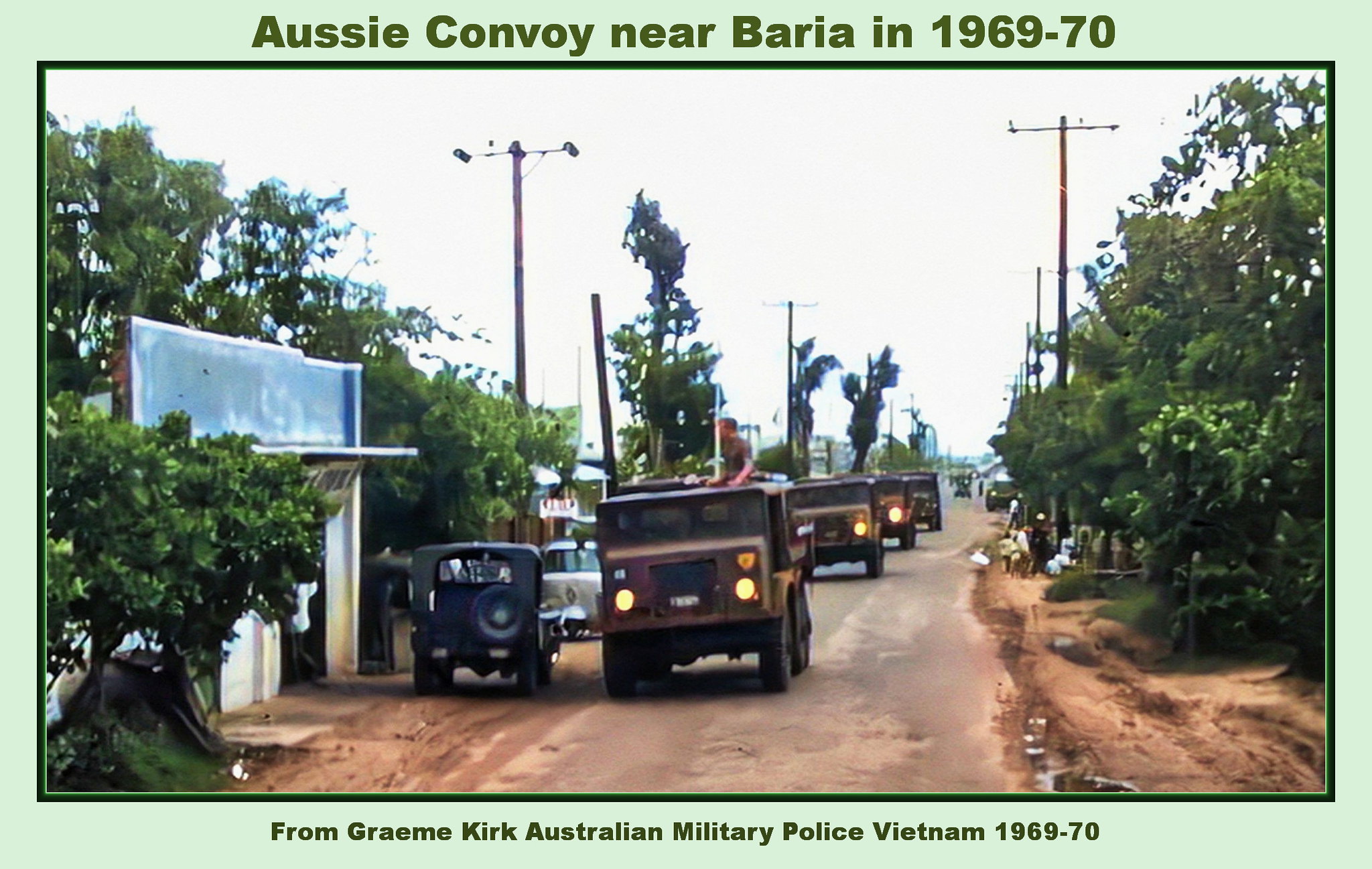The image depicts an Aussie convoy near Baria, Vietnam, between 1969 and 1970, as indicated by the green text on the mint-colored frame surrounding the picture. In the foreground, there's a medium-toned, reddish-brown dirt road lined with utility poles stretching into the distance, without visible power lines. The convoy consists of olive drab military trucks, each with headlights on. The lead truck has a white male with his sleeve rolled up, perched atop, seemingly scanning the area. Further back, additional trucks trail, diminishing in visibility. To the right of the road, there's a rich display of trees, indicative of a tropical setting. On the left, a significant white building with a light blue facade, possibly a store, stands framed by either concrete or wood. Adjacent to this building, a military Jeep, reminiscent of World War II, is parked, followed by another vehicle. Further left, more triangularly shaped trees recede into the background. The sky is uniformly white, suggesting an overcast or gray day, adding to the detailed and historical nature of the photograph. The bottom of the image is captioned in small green letters, attributing the photograph to Graham Kirk, of the Australian Military Police, active in Vietnam from 1962 to 1970.